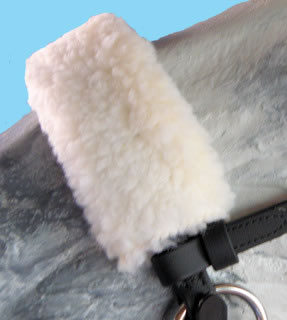This photo is an extreme close-up of a piece of horse equipment, focused on the horse’s face and nose. The horse is grey, and in the background is a vibrant blue color. The central feature in the image is a piece of white, wool-like fabric that gently loops across the horse’s nose. Attached to this fabric are black or dark brown straps, which connect to a metal ring, possibly brass. The intricate details and textures of the woolly fabric, straps, and metal ring indicate this might be part of a harness or reins used on a horse.